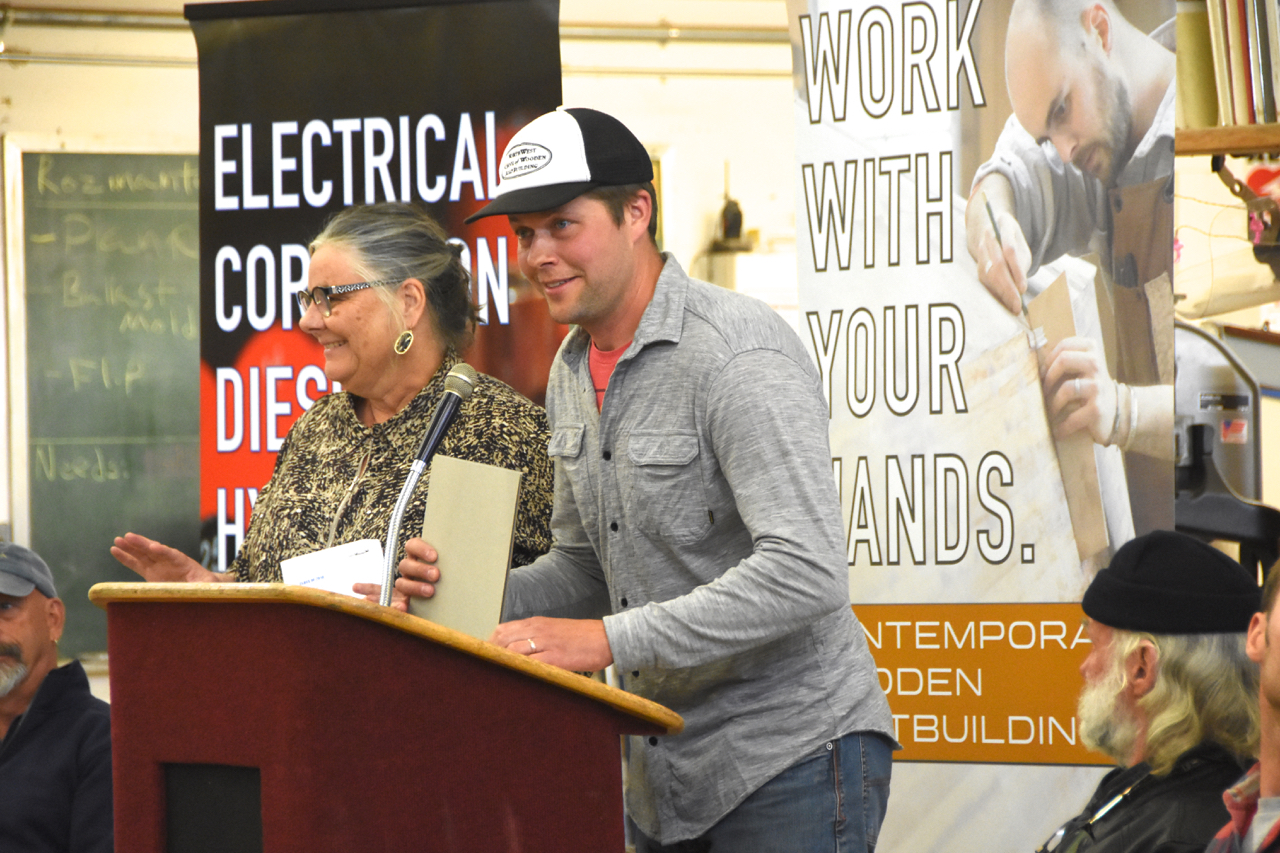In this detailed photograph, a casual scene unfolds at a podium crafted from dark and light brown wood. Two individuals stand behind it, engaged in an event likely set in a workshop or educational setting. On the right, a man in a long-sleeved gray shirt layered over a coral-colored shirt and blue jeans leans forward, smiling as he speaks into a black microphone on a silver stand. His white and black baseball cap slightly shades his eyes, and he clutches a booklet in one hand while resting the other on the podium. To his left, an elderly woman beams with her gaze directed off to the side. She wears glasses, her hair neatly tied back, a pair of green and yellow earrings, and a patterned shirt with light yellow and green hues. One of her hands is raised in an animated gesture, while the other holds a piece of paper.

The backdrop reveals a glimpse into the setting’s essence. A large freestanding poster boldly proclaims in white letters, "Work with your hands," accompanied by an image of a person engaged in woodworking. Additionally, partially obscured text hints at words like "electrical" and fragmented lines reading "COP," "D-I-E-S," and "H." This likely suggests a context involving manual skills and craftsmanship. Hints of a green chalkboard further blend into the background. Within the corners of the image, two older men with beards, possibly spectators in the workshop, provide additional context to the bustling environment.